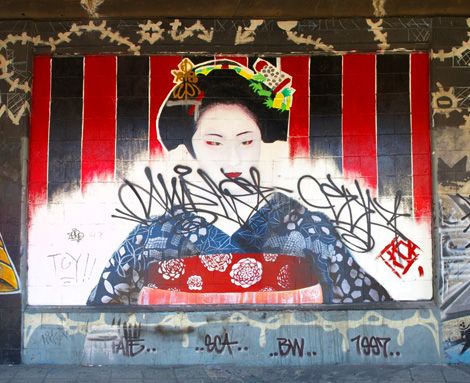This image depicts a mural of a classic geisha woman adorned in traditional attire, featuring a blue kimono with a red chest wrap, both embellished with floral patterns. Her hair is elegantly styled into a black bun, accessorized with intricate decorations, and her face is painted in typical white makeup with striking red lipstick. The mural's backdrop is composed of alternating vertical red and black stripes, merging into a semi-circular, white-washed border surrounding the figure.

However, the mural has been heavily graffitied, with a black marker's scribbles obscuring her chest and extending toward the viewer's right, accompanied by additional tags. To the left of the geisha, the word "TOI!" with two exclamation points is visible, while the bottom of the mural showcases a fishbone-like graffiti pattern including letters such as "BW" and a date "1997". The overall image has a slightly cramped composition, appearing as a photograph of a poster or a mural in an urban setting.